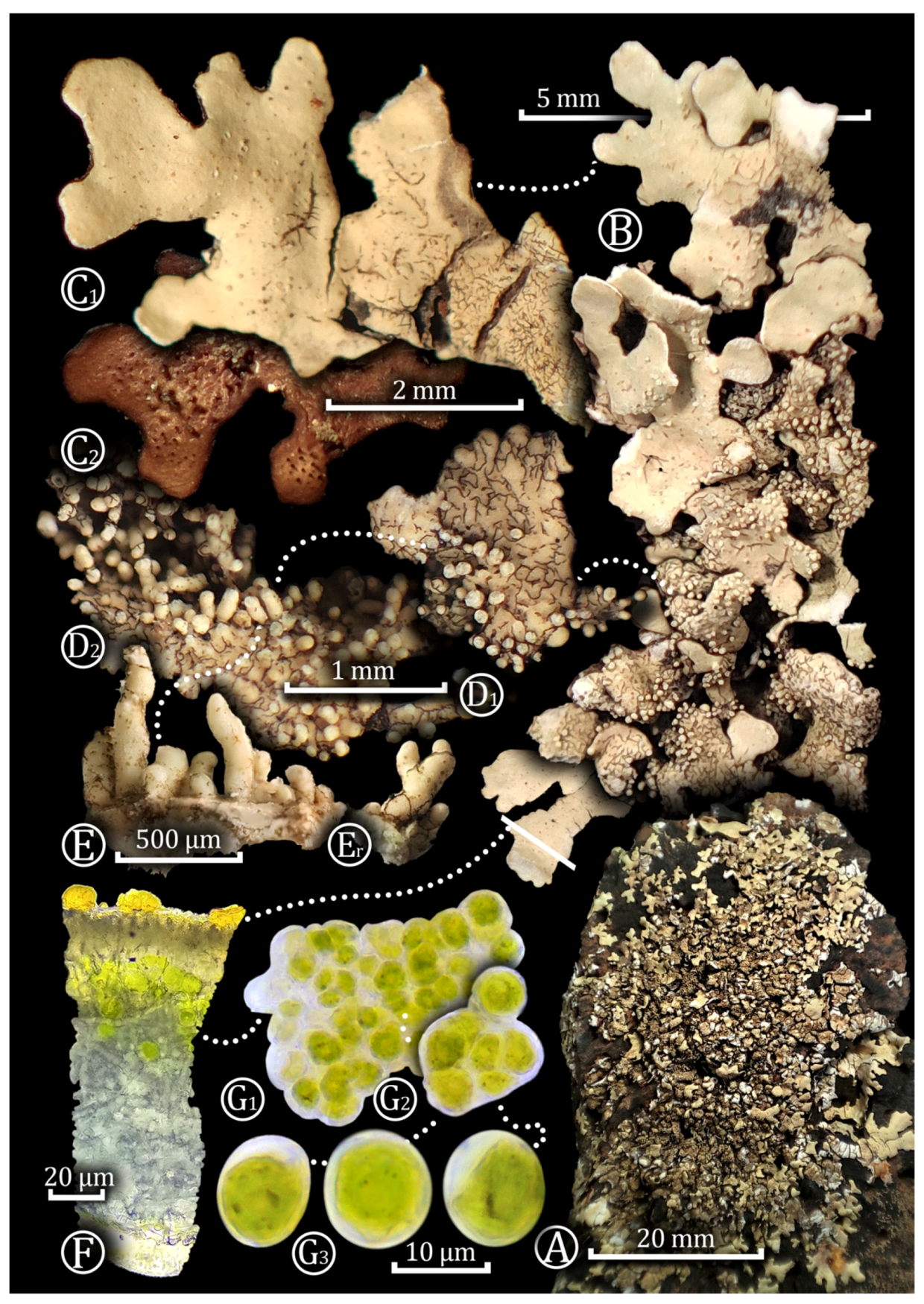This vertically rectangular image features a vibrant, colorful poster set against an intense black background. The poster showcases various types of objects that appear to be different forms of fungi or mushrooms, possibly viewed under a microscope. The top section displays flaky, light tan fungi, with similar beige and tan flaky specimens lining the entire right side. The left side hosts darker brown fungi at the top, transitioning to lighter tan and beige in the center, with some resembling tiny, upright fingers. At the bottom left, white circular shapes with green centers are visible, accompanied by a column-shaped fungus on the very left, which is white at the base, gray in the middle, and greenish-yellow at the top. Each type of fungus is meticulously labeled with designations such as A, B, C, C2, D, D1, D2, E, E1, G1, G2, G3, and F. The image also includes an array of measurements to illustrate size, ranging from 1 millimeter to 20 millimeters and even finer measurements in micrometers for the smaller, green circular spots.